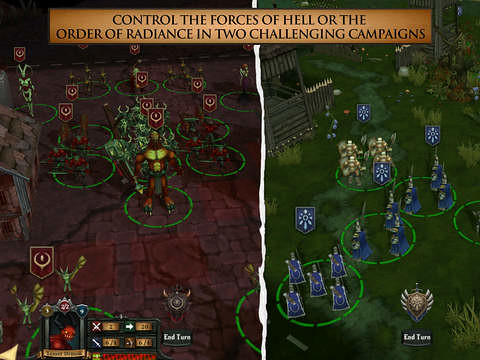The image depicts a promotional poster for a video game, artfully torn into two halves and reassembled, creating a dramatic and intriguing visual effect. Bold text across the top proclaims, "Control the forces of Hell or the Order of Radiance in two challenging campaigns." On the left side of the image, the background is a deep, ominous red, accentuated with glowing green circles. This side features shadowy, indistinct figures that may represent characters or warriors, and emblazoned shields that hint at conflict and combat. On the right side, the background shifts to a more verdant green, maintaining the green circles but introducing blue shields that contrast with the red side. Here, a rustic log cabin stands out amid the ethereal backdrop, suggesting a different setting or strategy element for the campaign. Together, the two halves promise diverse gameplay experiences, one dark and menacing, the other verdant and fortified.